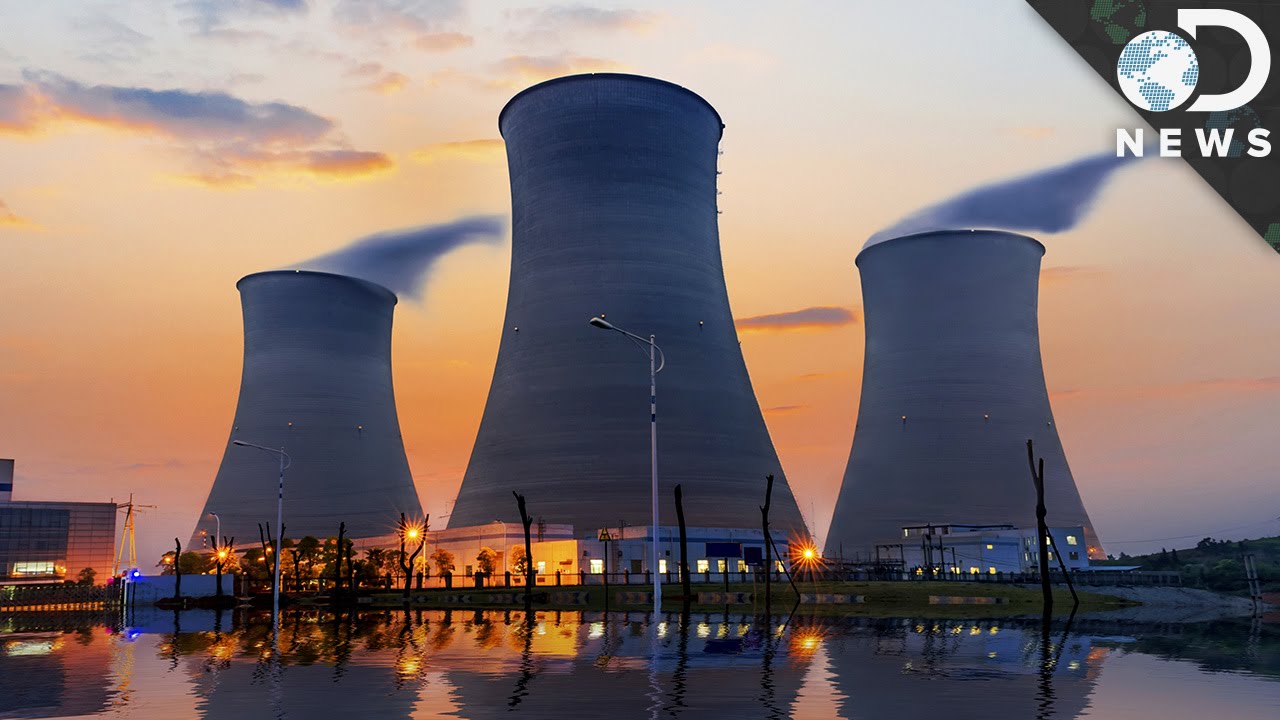The newspaper photo showcases a nuclear plant at twilight or dawn, identified by the prominent "D News" logo in the upper right corner, featuring a capital D and a small globe. Central in the image are three cooling towers of nuclear reactors, with the largest in the center and two smaller ones flanking each side. The twilight sky paints a dramatic backdrop with hues of orange and red, accentuated by clouds seemingly fuming from the towers. A serene body of water lies in the foreground, capturing reflections of the cooling towers and amplifying the dark blue and purple tones of the scene. Surrounding the plant are several modern buildings, possibly labs or warehouses, alongside a few palm trees, hinting at a warm climate. A small structure in the bottom left corner and bordering streetlights add to the industrial setting. The photo, with its blend of natural beauty and industrial might, offers a striking and modern portrayal of the nuclear facility.